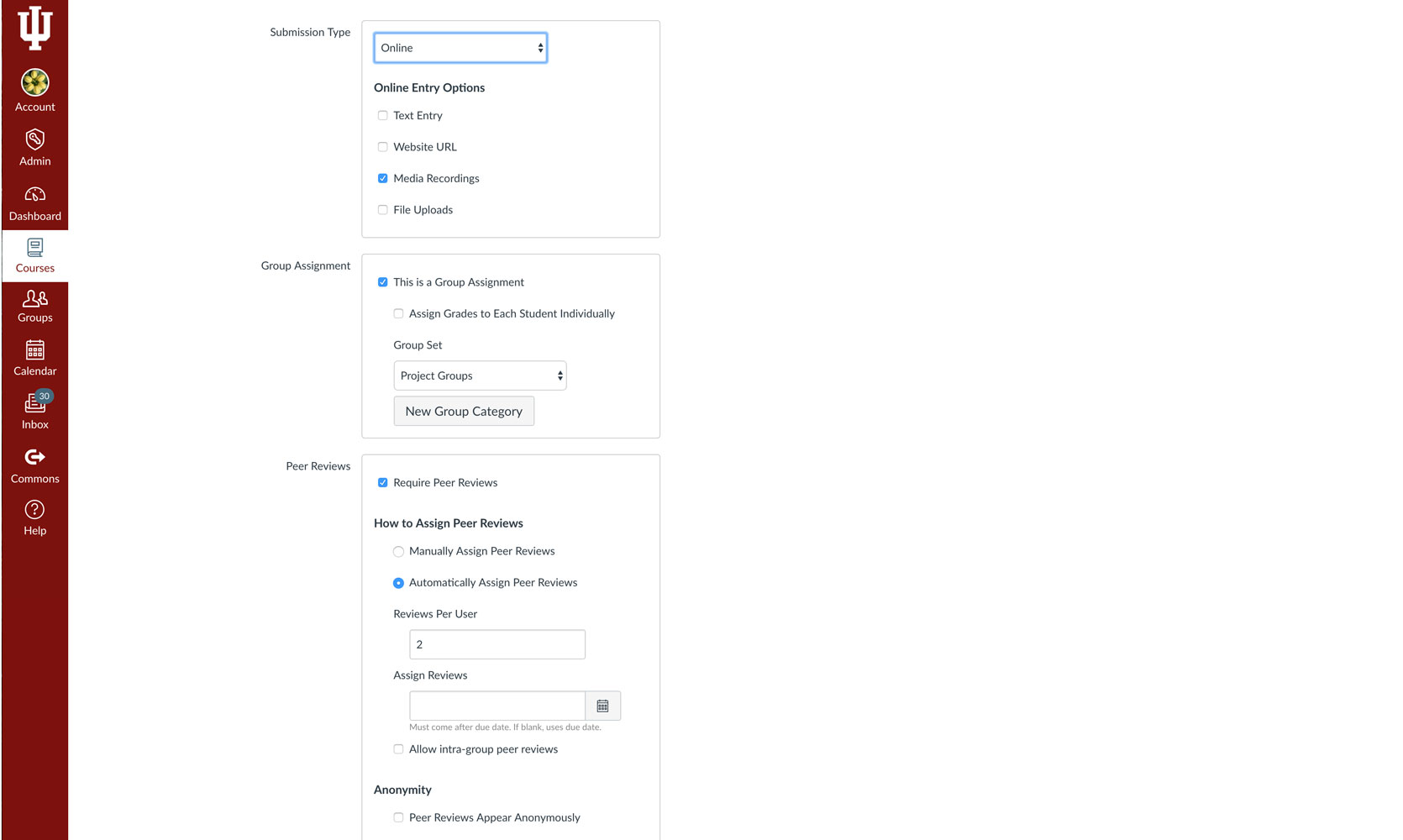The image showcases a digital form interface set against a white background, featuring a distinctive red vertical bar on the left side for emphasis. Within this interface, there are three prominent white rectangles, each designed to specify various elements of an assignment submission process.

The first rectangle is titled "Submission Type." This section is highlighted with a blue box labeled "Online" and encompasses multiple online entry options including "Text Entry," "Website URL," with each of these individual options being accompanied by checkboxes for user selection. Additional available options for submission include "Media Recordings" and "File Uploads," each also accompanied by a checkbox to enable these features.

Below the submission type selections, there is a segment dedicated to "Group Assignment." Here, there is a checkbox labeled "This is a Group Assignment," offering the functionality to assign grades to each student individually. Additionally, the section features a label "Group Set," followed by "Project Groups," and a gray-colored rectangle containing the text "New Group Category." 

The final segment of the interface pertains to "Peer Reviews." This section provides a checkbox titled "Require Peer Reviews," accompanied by a directive on "How to Assign Peer Reviews." Within this, users have the option to manually assign peer reviews, alongside a checkbox specifically for this feature.

Overall, the detailed and structured interface aims to facilitate a comprehensive and customizable assignment submission and review process.